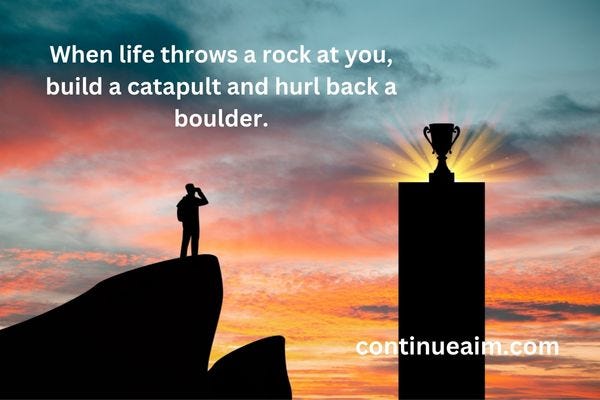The image captures a stunning sunset with a gradient of blues, pinks, and oranges melting into a brilliantly glowing yellow horizon. In the foreground, on the left-hand side, a black silhouette of a man stands resolutely on a rock, his hand shading his eyes as he gazes intently at a trophy perched on a tall plinth across from him. Behind the trophy, radiant sunbeams burst outward, emphasizing its significance and adding a dramatic flair. On the upper left side, a motivational quote in white letters reads, "When life throws a rock at you, build a catapult and hurl back a boulder." At the bottom right, the website "ContinueAIM.com" is displayed in white text, subtly blending with the serene yet powerful scene.